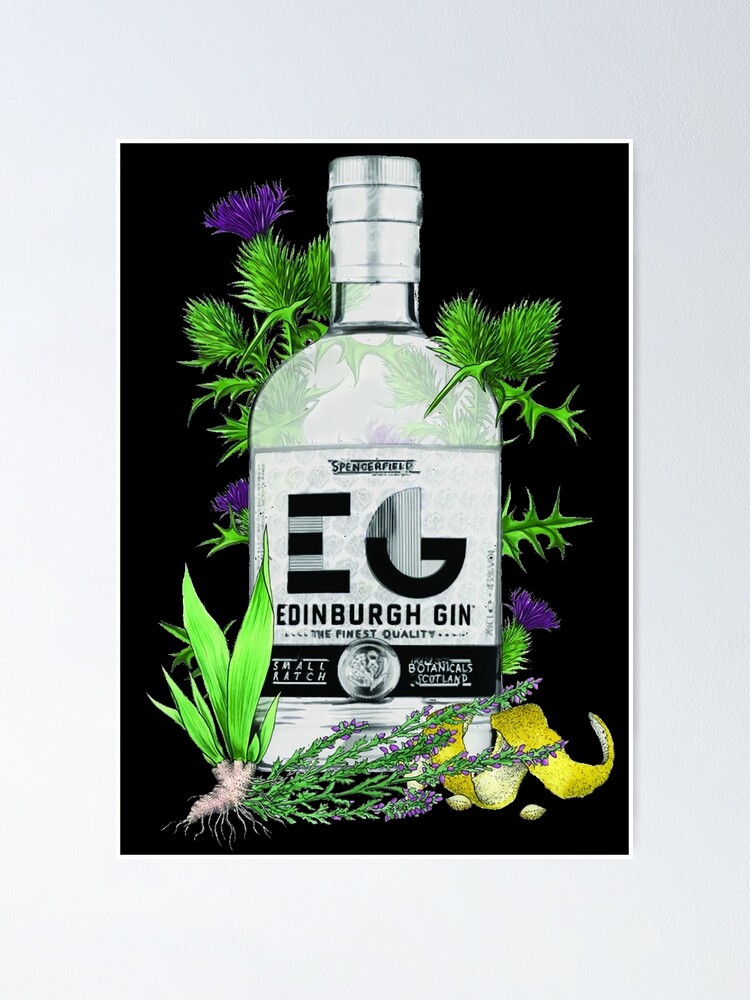The image showcases a white bottle of Edinburgh Gin set against a solid black background. The bottle prominently fills the majority of the frame, featuring the brand name "Edinburgh Gin" with the logo "EG" and the phrase "the finest quality" in small text beneath it. Encircling the bottle are various green leaves and purple flowers, adding a natural, botanical aesthetic. A silver cap tops the bottle, which is further adorned with plants and yellow lemon peels near the bottom right. The artwork appears to be digitally crafted, resembling high-quality graphic design, and is framed in white, giving it an elegant, display-worthy appearance.